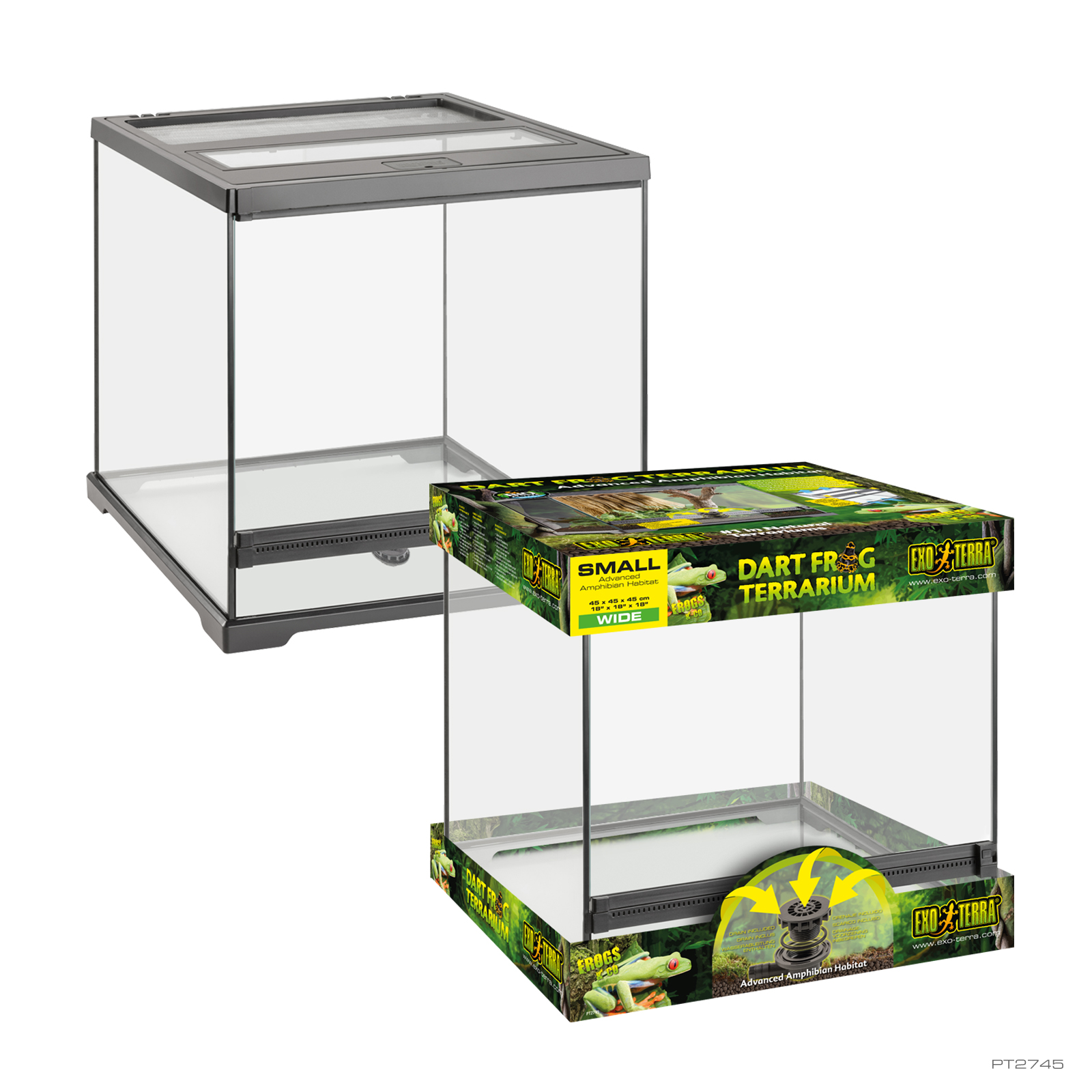The photograph displays two terrariums positioned at an angle, with one located in front of the other. The terrarium in the back is a clear, square structure with glass panels and a distinctive black plastic frame. It features a segmented gray plastic lid and a matching gray base with small feet. The terrarium in the front is identical in structure but remains encased in its packaging. The packaging includes green cardboard covers at both the top and bottom. The top cover prominently features the text "Dart Frog Terrarium" along with "small" in black text on a yellow background and "small wide" in white on green. The upper section also includes images and illustrations of frogs. The bottom cover shows how to adjust the terrarium and includes additional images of frogs, with the "Exo Terra" logo in the lower right corner. These visual elements provide a comprehensive look at the terrarium, both packaged and unpackaged.